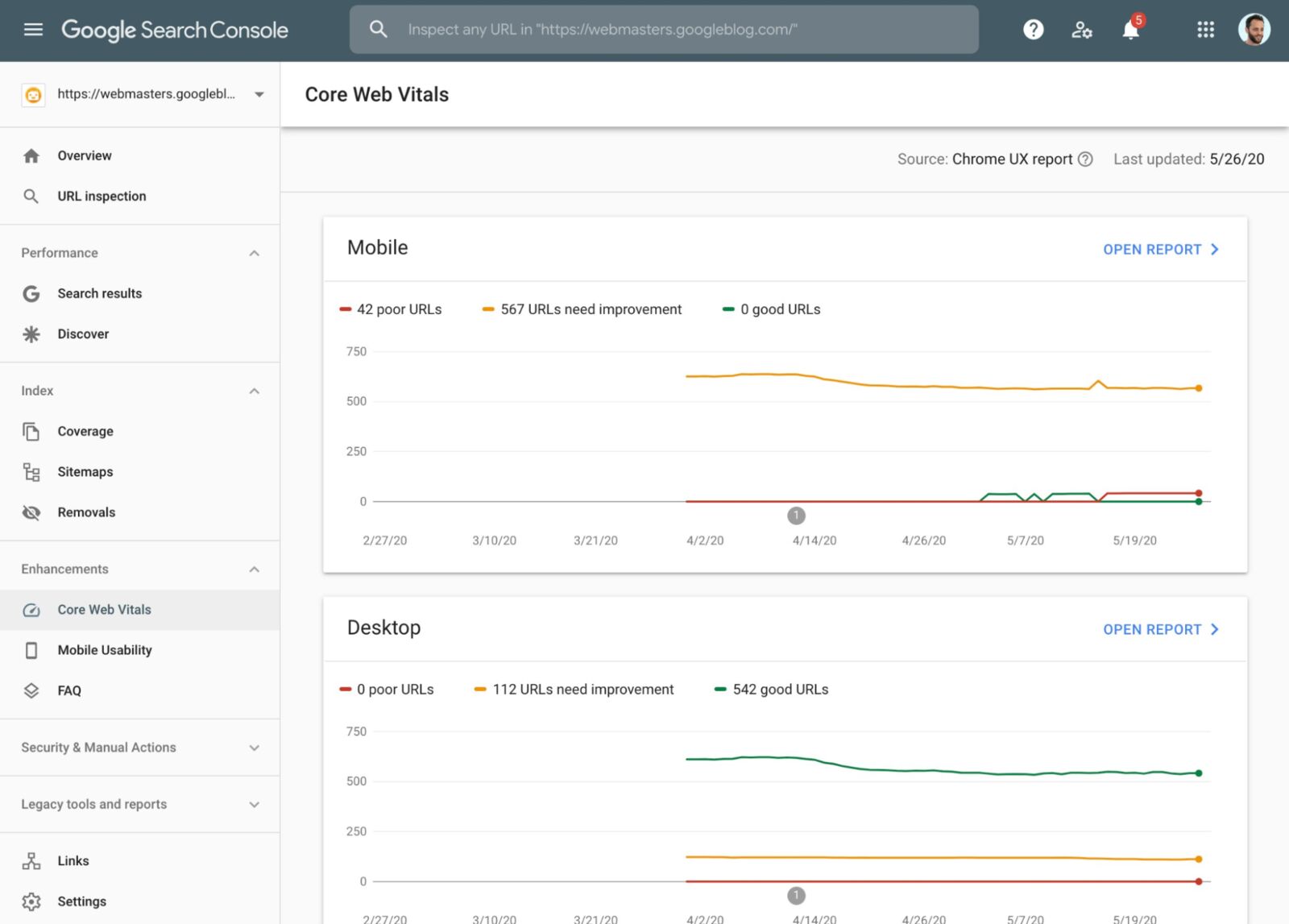The image displays the Google Search Console interface. At the top, a gray bar spans the width of the screen. On the far left of this bar, there is a "List" button. To the right, the text "Google Search Console" is prominently displayed. Centrally aligned on the top bar is a search bar, accompanied by a help button, a user settings button, and a notification center icon. Towards the far right, there is a user icon or profile picture.

Descending along the left side of the interface is a navigation panel that includes a website link with a drop-down menu. Below it, the menu lists various sections: "Overview," "URL Inspection," and a "Performance" tab that includes "Search Results" and "Discover." Further down, under the "Index" section, there are options such as "Coverage," "Sitemaps," and "Removals." The "Enhancements" tab features options for "Core Web Vitals," "Mobile Usability," and "Frequently Asked Questions." Additional sections include "Security and Manual Actions," "Legacy Tools and Reports," "Links," and "Settings."

In the central pane, the interface displays the "Core Web Vitals" section, featuring two graphs—one for mobile performance and another for desktop performance. Both graphs have accompanying "Open Report" buttons for further details.